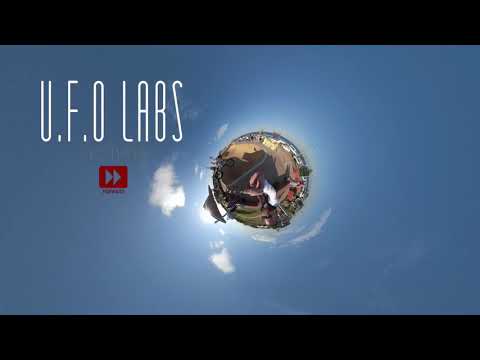The image features a computer-generated, panoramic view that creates the illusion of a tiny, spherical planet against an expansive blue sky scattered with a few white clouds. The small planet showcases a variety of details including green landscapes, rocky textures, roads, and small buildings, giving it a realistic yet fantastical feel. Encircling this miniature world, the sky and clouds almost seem to rotate around it. Positioned on the left side of the sphere, a spaceship-like object can be seen orbiting around the 'planet.' The image is framed by horizontal black bars, resembling widescreen movie borders. In the upper left corner, prominent white uppercase text reads "UFO Labs," accompanied by a small red box containing two transparent, fast-forward-style arrows.